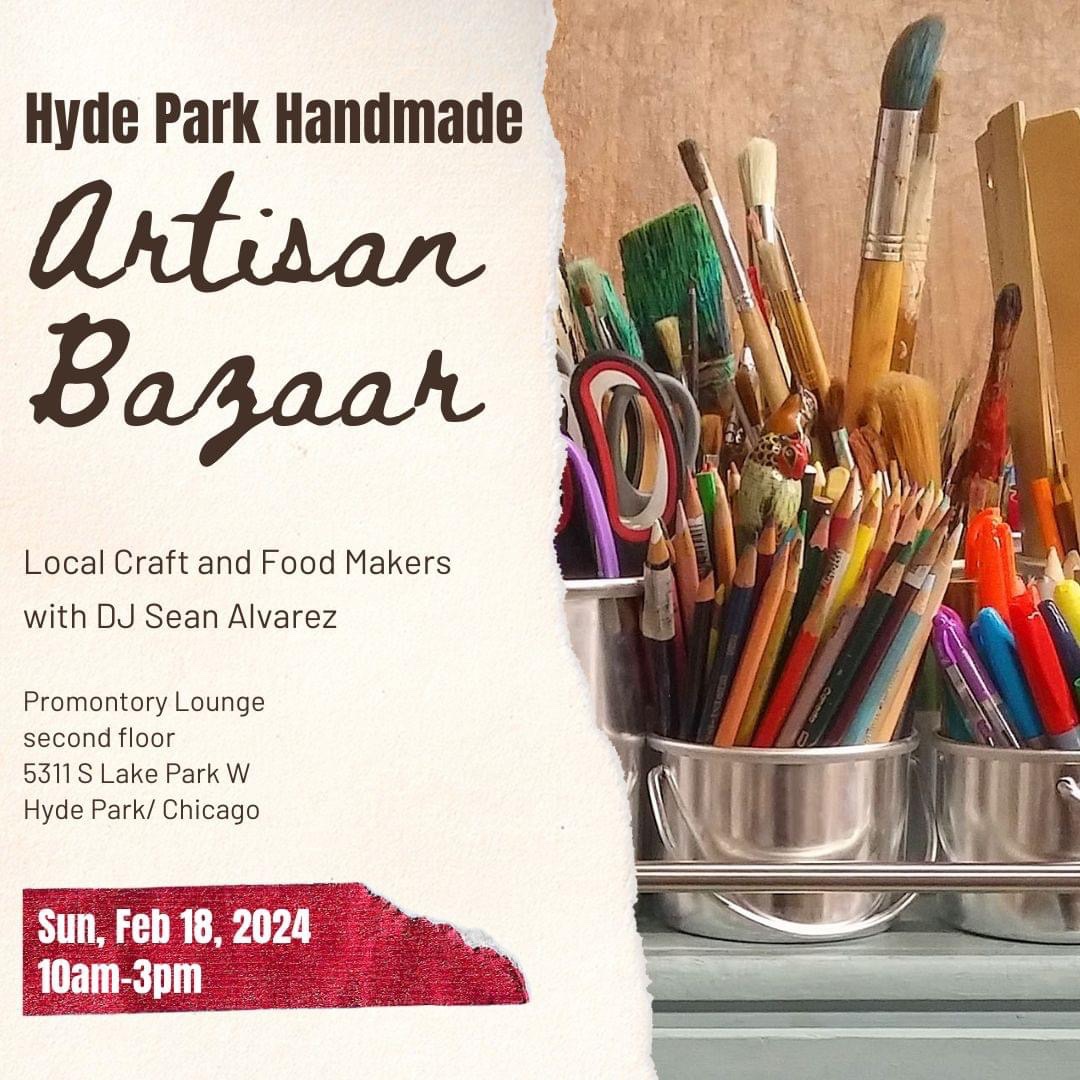This advertisement for the Hyde Park Handmade Artisan Bazaar prominently features art supplies on the right side, with several small metal buckets. The foremost bucket contains an array of colored pencils, while the adjacent bucket is filled with various colored markers. In the back row, the leftmost bucket holds at least two pairs of scissors and other indistinct items, and the next bucket showcases a collection of paint brushes in various sizes. The left half of the flyer is tan and contains text. At the top, it reads "Hyde Park Handmade" in brown, followed by "Artisan Bazaar" in large cursive. Beneath that, in regular font, it states "Local Craft and Food Makers with DJ Sean Alvarez." It also provides the location details: "Promontory Lounge, second floor, 5311 South Lake Park W, Hyde Park, Chicago." The bottom features a torn-paper effect revealing the event date and time in a red rectangle: "Sunday, February 18, 2024, 10 a.m. to 3 p.m."